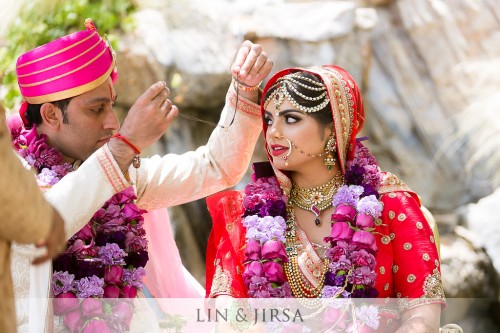An evocative photograph captures an Indian wedding ceremony, presumed to feature the couple named Lin and Jirsa as indicated by the text on the image. The groom, positioned on the left side of the photo, wears an elaborate pink and gold turban paired with a whitish-pink long-sleeved shirt. He drapes festive layers of pink and purple flower wreaths around his neck. With his left arm raised, he appears to be holding a necklace above the bride's head. The bride stands to his right, adorned in an opulent red and gold dress with a hood. Her look is completed with a dazzling array of gold jewelry, including various long and tight necklaces, earrings, intricate headwear, and a nose ring. She, too, wears layers of pink and purple flowers around her neck. The setting suggests an outdoor gathering in nature, enhancing the regal and joyous atmosphere as the couple, looking radiant and ready to embark on their new journey together, participates in this sacred ritual.